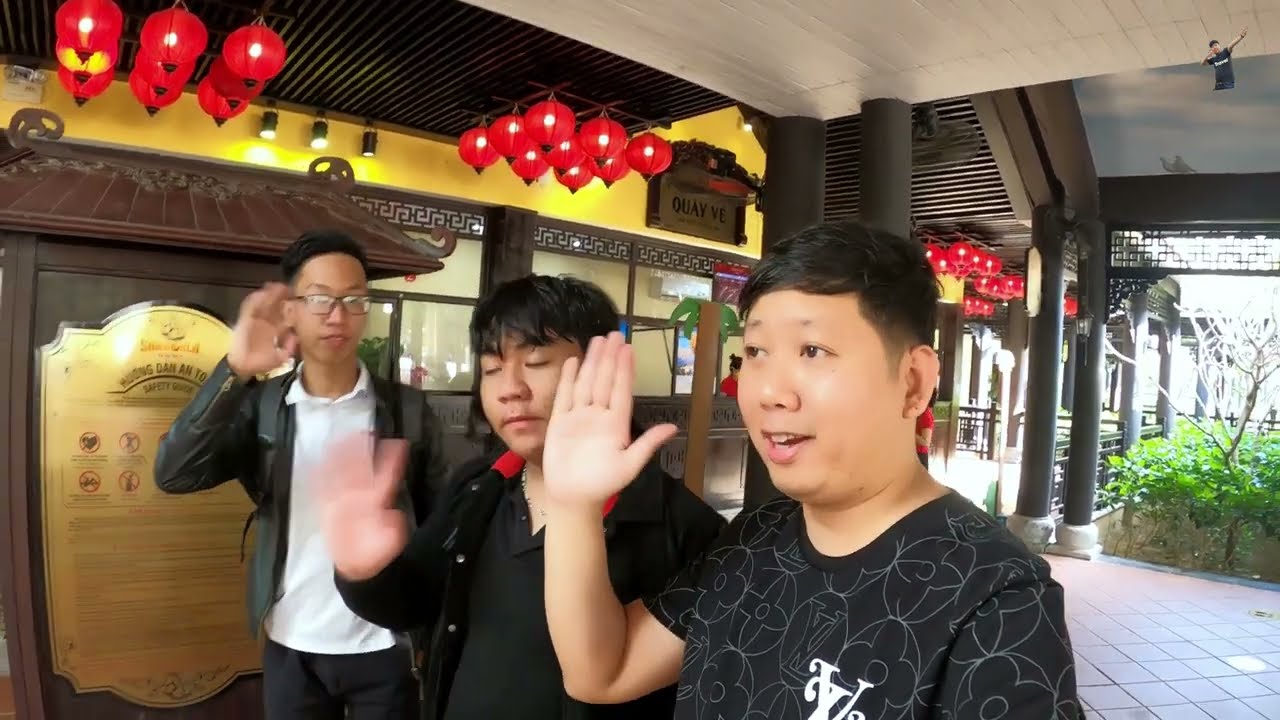The photograph features three teenage males of Asian descent, possibly Cambodian, standing under an ornate wooden ceiling with white beams. They all have light brown complexions and black hair. The young man on the right is gazing to the left and wearing a black shirt adorned with white details resembling flower petals and a Louis Vuitton logo. The central figure wears a black jacket with a red collar, over a partially open black shirt. The leftmost young man, who sports glasses, is clad in a green jacket with zippers over a white shirt and black pants.

All three boys have their hands raised in various gestures—some appearing to wave, indicated by the blurriness of their motions, and one holding his hand straight up as if signaling to stop. The setting appears to be the covered entrance of a building, potentially a Chinese restaurant, suggested by the decorative red lanterns hanging from the structure and details that resemble typical Chinese architectural elements.

In the background, there are brown wooden pillars with white bases supporting the canopy. A yellow wall stands out behind some garden elements and lights encased in red globes arranged in patterns. Signage can be seen on the right, likely explaining the purpose of the facility, and another plaque is mounted on the yellow wall beside a door. The floor is tiled in light brown, completing the scene's intricate backdrop.